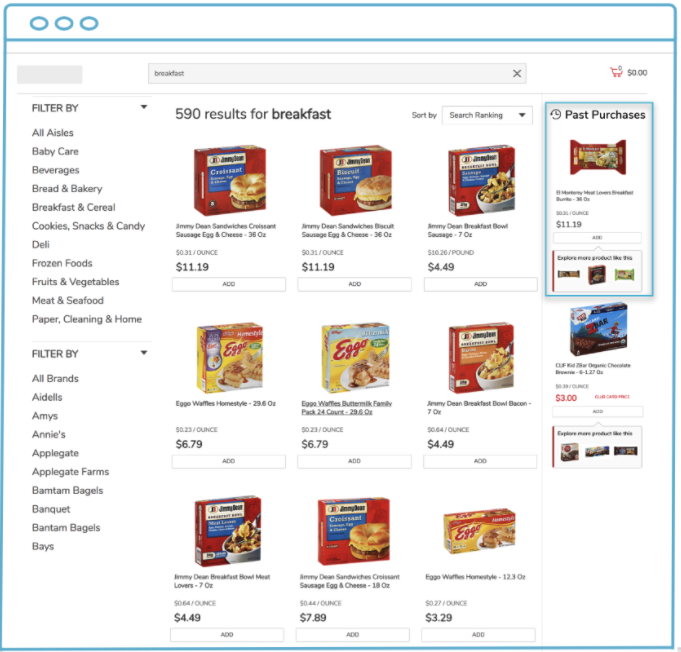The image is a screenshot from a website, featuring a turquoise, blue-based border outlining the entire perimeter. At the top, there is a prominent white banner containing three oval icons aligned side by side. Below this banner, a gray search bar displays the text "breakfast." Adjacent to the search bar, a red shopping cart icon indicates "$0" and "zero items in the cart." 

On the left side of the image, a filtering section labeled "Filter By" provides various store categories and allows further refinement by brands. 

In the main content area, the center and right sections showcase the search results. An informative header states "590 results for breakfast," accompanied by a dropdown menu for verifying search rankings. The search results are displayed in a grid with three rows and three columns of breakfast items. 

On the far right, there's a section labeled "Past Purchases," highlighted by a blue-trimmed box, offering quick access to previously bought items.